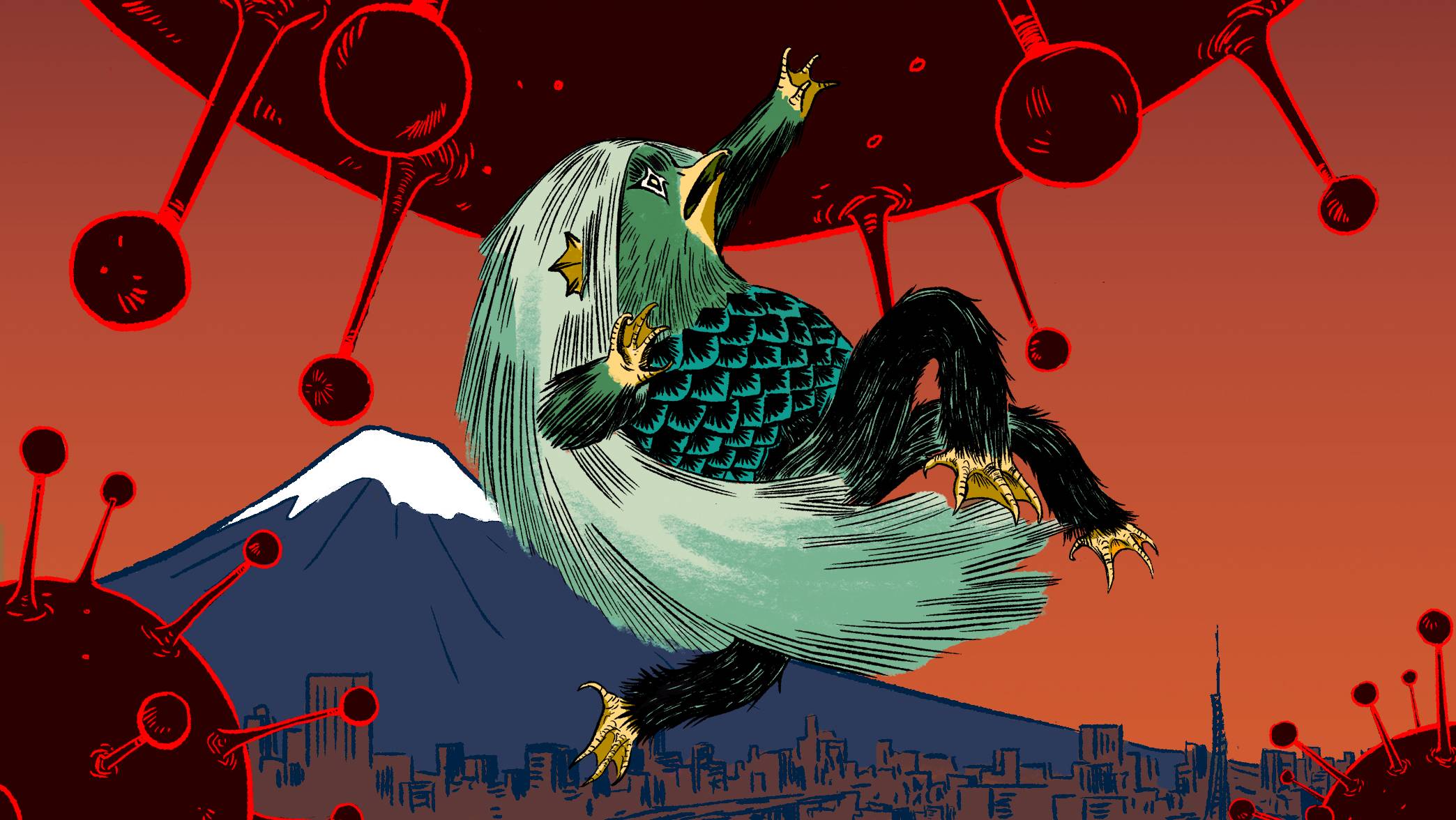This intriguing landscape-oriented artwork appears to be a computer-generated illustration, featuring a striking mythical creature as its central motif. The creature, a chimeric amalgamation with elements resembling both a bird and an aquatic animal, stands out vividly. It has a bird's beak, three black legs with webbed feet, and bird-like claws. Its body is covered in dark green, feather-like fur, complemented by long lime green hair cascading down its back. The creature also features unique fins for ears and webbed, alien-like hands, giving it an otherworldly appearance.

The backdrop showcases a detailed scene of a cityscape with skyscrapers, set against the imposing silhouette of the snow-capped Mount Fuji. The twilight-red sky, transitioning into burnt orange hues, adds a dramatic tone to the composition. Surrounding the mythical being, there are three large, dark red spherical viruses. Each virus is ominously spiked and reminiscent of bacteria, floating around the periphery of the scene. One of these virus-like forms is conspicuously placed in the bottom right corner, emphasizing the surreal juxtaposition of elements within this artwork.